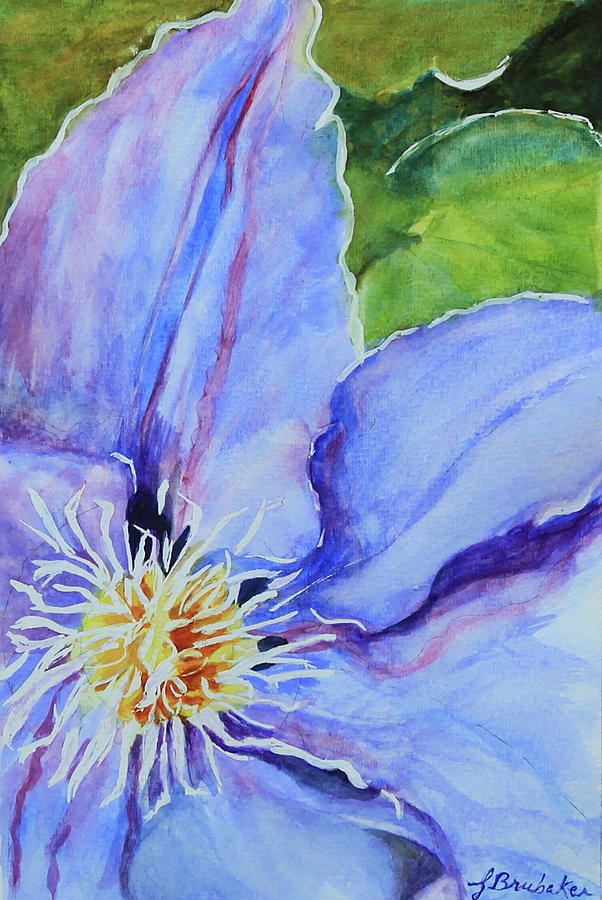The artwork in the image is a detailed close-up of a single flower, predominantly blue with shades of purple and pink throughout the petals. The flower's center is a striking yellow with orange accents, featuring delicate white tendrils protruding from it. The petals, which dominate the image, are intricately colored with lines of pink and dark blue, blending seamlessly into lighter shades, giving the flower a mesmerizing, almost ethereal quality. The petals fill most of the frame, with the exception of the top right corner, where some light green leaves, streaked with dark green, extend into the space, providing a contrasting background to the vivid flower. The image, resembling a watercolor painting, contains the artist's signature in the bottom right corner, written in blue ink or paint, reading "Jay Brubaker." This signature confirms the artwork's authenticity, adding a personal touch from the artist. The composition suggests that the flower is situated in a natural setting, complemented by green foliage beneath and around it.